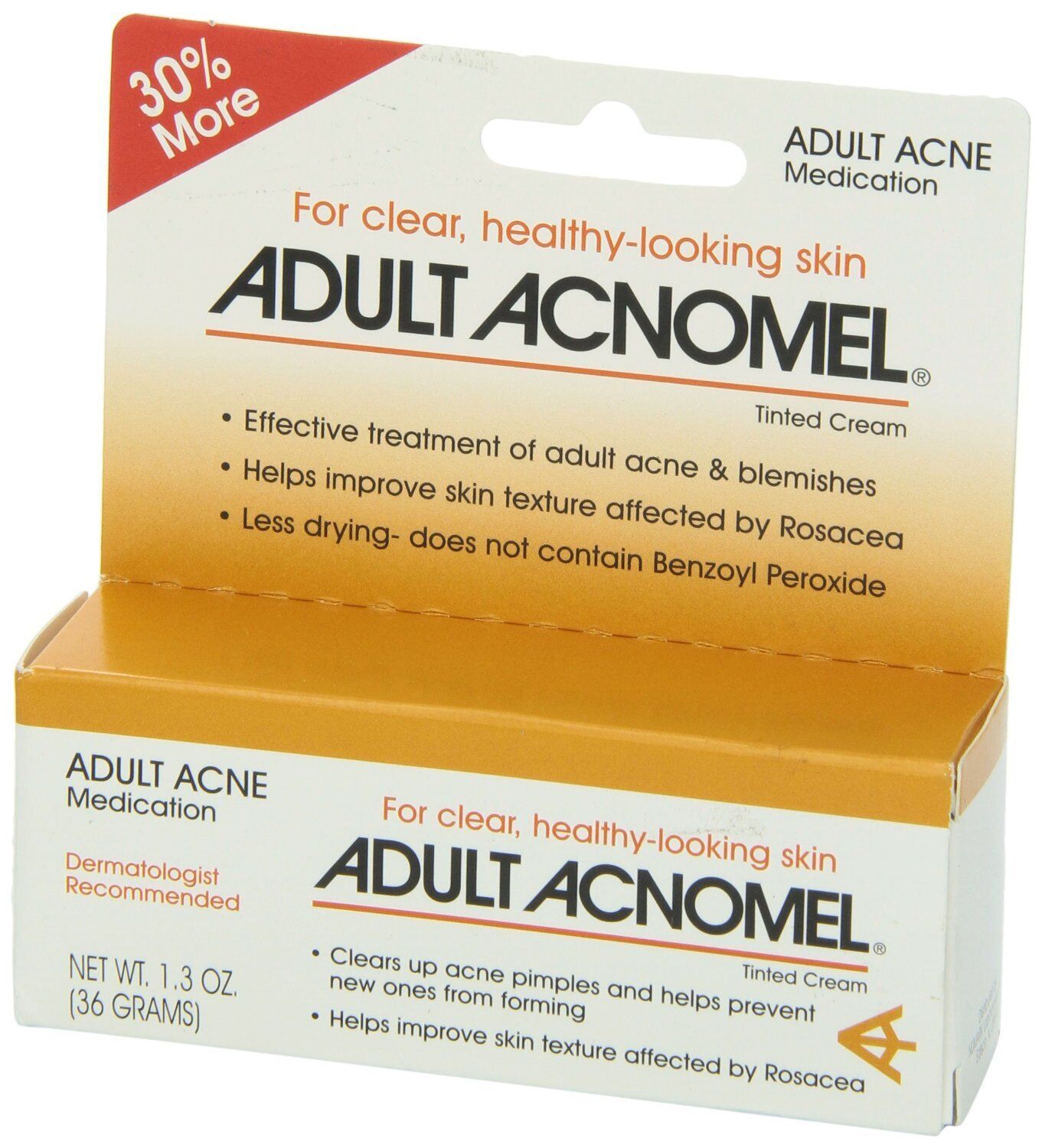The image depicts a color photograph of a product package for "Adult Acnomel Tinted Cream." The box, angled diagonally and facing the bottom left, has a predominantly white background that fades into orange or yellow at the top. In the top left corner, there's a prominent red triangle with the text "30% more" in white. On the front, the text "For clear, healthy-looking skin" is written in orange, followed by "Adult Acnomel Tinted Cream" in bold black letters. The top right corner states "Adult acne medication" in black text. Beneath the main text are three bullet points: "Effective treatment of adult acne and blemishes," "Helps improve skin texture affected by rosacea," and "Less drying, does not contain benzoyl peroxide.” Additionally, there’s an insignia resembling a sideways ‘A’ blended with a left-facing arrow. The bottom section mentions "Dermatologist recommended," and notes the net weight as 1.3 ounces or 36 grams. The packaging includes a hook for hanging on a retail display, and it appears to contain a tube of the product inside.